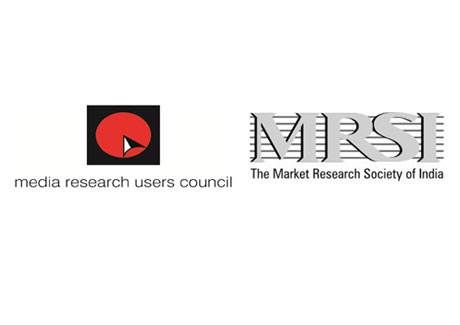The image presents two distinct logos side-by-side, with no border or specific orientation separating them. On the left, the logo is composed of a black square box featuring a red circle slightly off-center. Within the bottom right quadrant of the circle, an arrow outlined in black points upward toward the center, with the left half of the arrow in white and the top half in black. Below this icon, in small dark gray text, reads "Media Research Users Council." 

To the right, the second logo displays the acronym "MRSI" in a 3D capital letter font. The letters are light gray with a black background providing a shadow effect. Horizontal gray lines serve as a backdrop to the text. Beneath "MRSI," small bold black text states, "The Market Research Society of India."